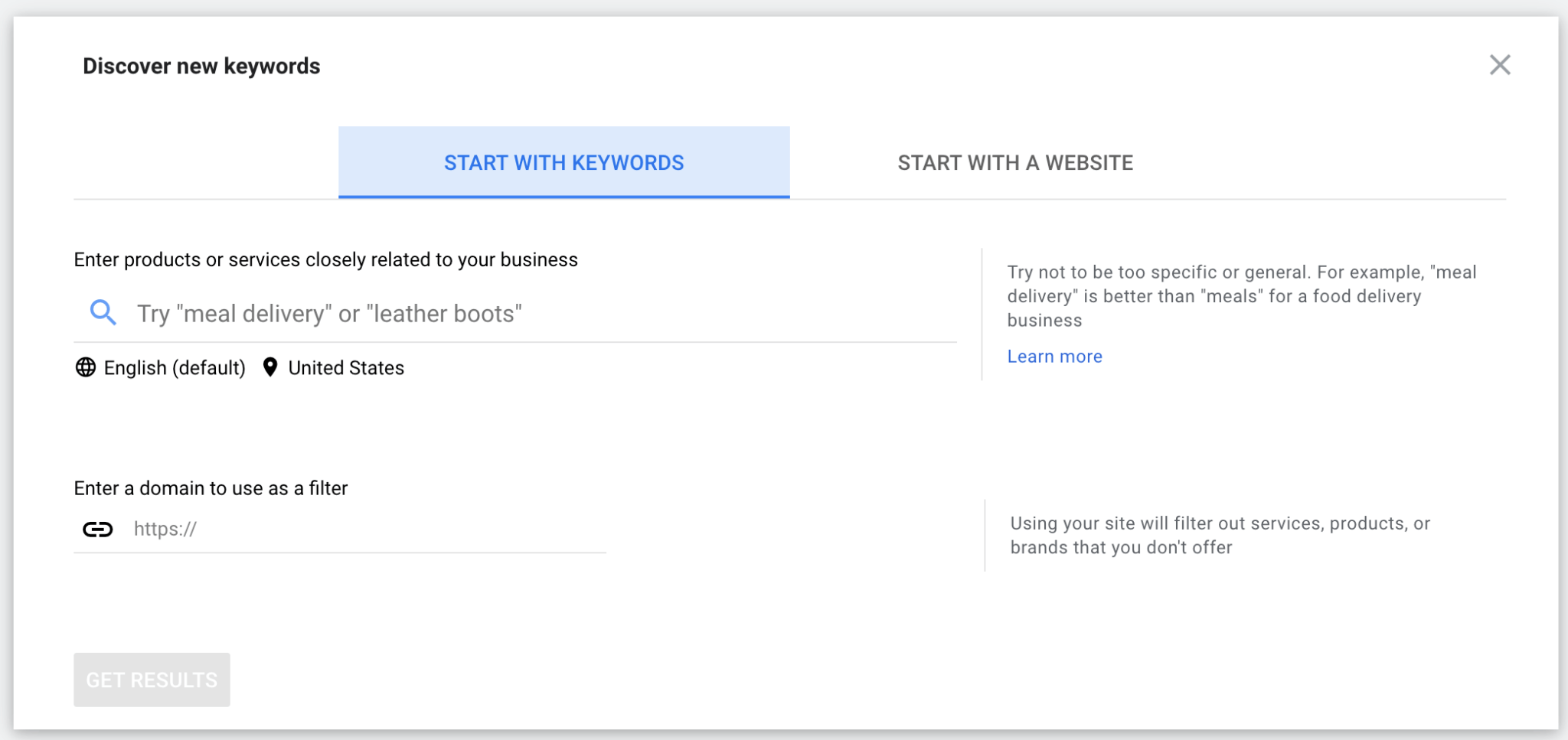This is a screenshot of a pop-up menu with a white background. In the upper left corner, black text reads "Discover new keywords." On the upper right corner, a small gray "X" allows users to close the pop-up menu. Below this header, there are two selectable options: "Start with keywords" and "Start with a website." The selected option is "Start with keywords."

A thin black line separates the options from the next section, which instructs users to "Enter products or services closely related to your business." Directly below this prompt, there is a search field accompanied by a blue magnifying glass icon. The placeholder text within the search field, in gray font, suggests examples like 'meal delivery' or 'leather boots.'

Further down, black text indicates "English (Default) - United States." Below this, another instruction in black font says, "Enter a domain to use as a filter." A corresponding input field begins with "https://", prompting the user for a web address.

In the lower left corner of the pop-up, a grayed-out rectangular button with white text says "Get results." To the right of this button, additional information is provided in gray font.